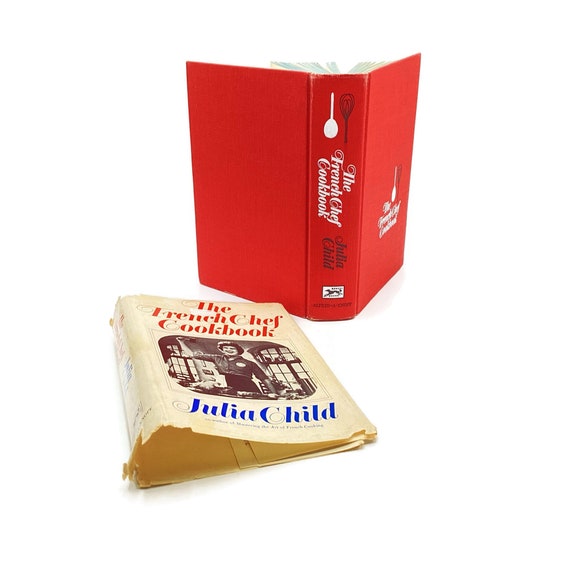The image features a photograph of an upright book with a red jacket, positioned centrally against a plain white background. This book, "The French Chef Cookbook" by Julia Child, is detailed in white cursive letters both on its spine, along with illustrations of a white spoon and a black spatula, and on the front cover. The red book is paired with its removed, slightly tattered beige dust jacket. The jacket displays the book's title, "The French Chef Cookbook," in red and the author’s name, Julia Child, in blue at the bottom. Between the title and author name is a black-and-white photograph of Julia Child standing in a kitchen. The red book is opened to some extent, revealing glimpses of its pages at the top. This setting with the focus on books aligns with themes of reading and culinary arts.